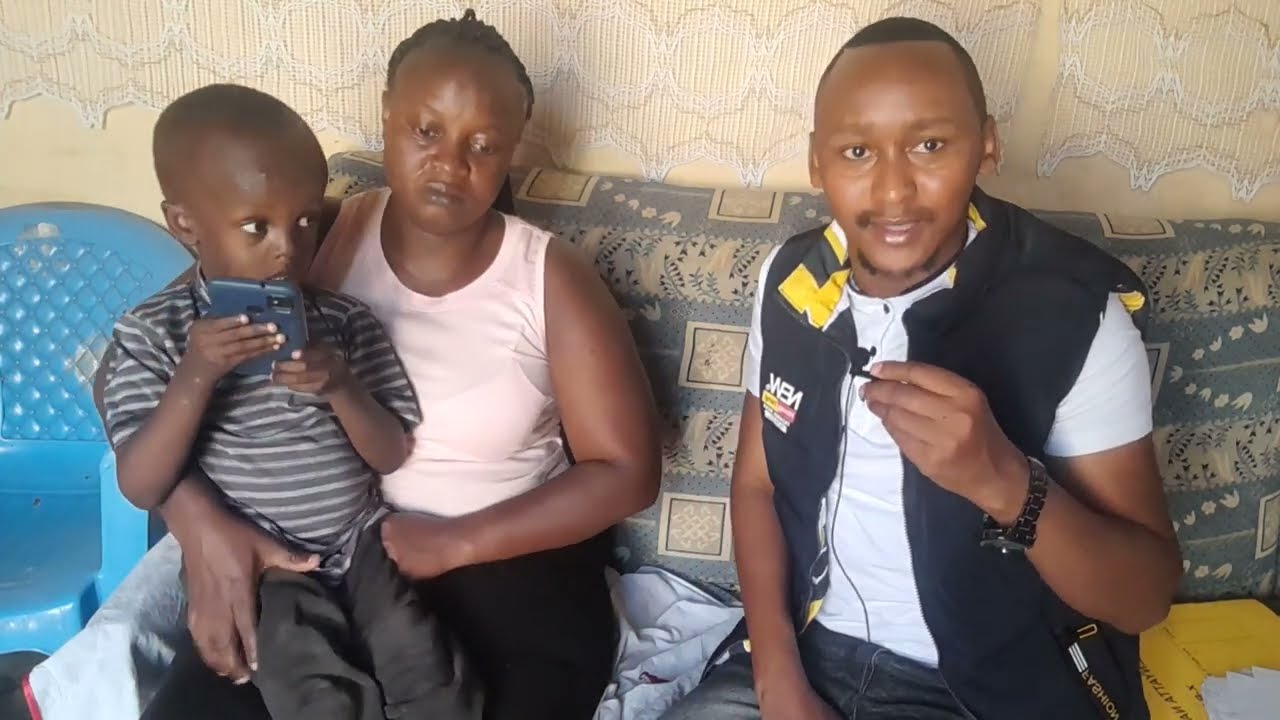In this photograph, three individuals—a woman, a man, and a child—are seated on a grey and cream-colored sofa against a peach-colored wall adorned with a net-like cloth. The woman, positioned on the left side, is wearing a pink t-shirt and black pants, and appears somewhat sad as her gaze is directed slightly downward. She holds a young boy on her lap, who is dressed in a grey shirt with white stripes and grey pants, holding a blue mobile phone while looking off to the right. To the woman's left, a blue plastic chair is visible. On the right side of the sofa sits a man, wearing a white t-shirt under a blue-black jacket and black pants. He has a watch on his left wrist and is holding a microphone in his left hand, seemingly speaking. The back of the sofa has some designs, and to the man's right lies some mail, including an envelope and a few papers. The overall scene suggests a candid moment captured during what might be an interview or a casual family interaction.